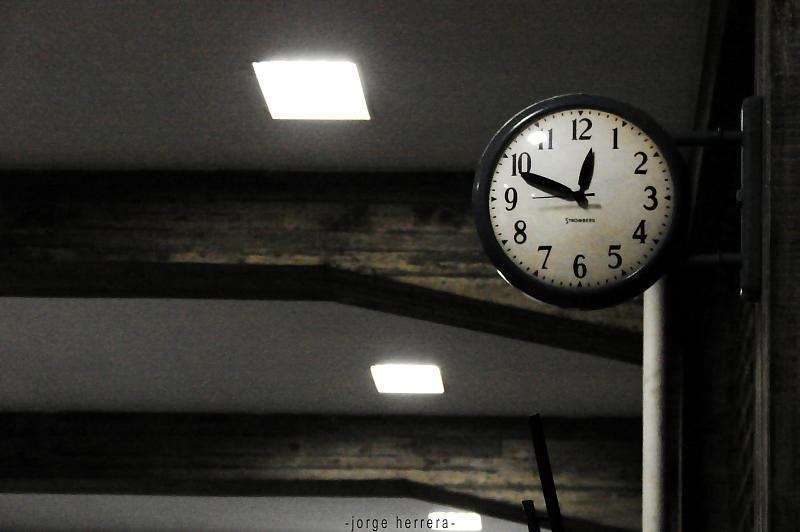The indoor photograph captures an architectural ceiling adorned with three light fixtures. Massive wooden beams run horizontally, intersecting the area between the light fixtures, giving the ceiling a rustic charm. To the right, a wall stretches from the top to the bottom of the image. A metal pole stands vertically in front of this wall, and attached to the pole is a round black clock. The face of the clock is round and white, featuring black numbers from 1 through 12 and minute markings in between. The black clock hands point to 12:49, and beneath the hands, there is an indistinguishable word. At the bottom center of the photo, the name "Jorge Herrera" is prominently displayed.